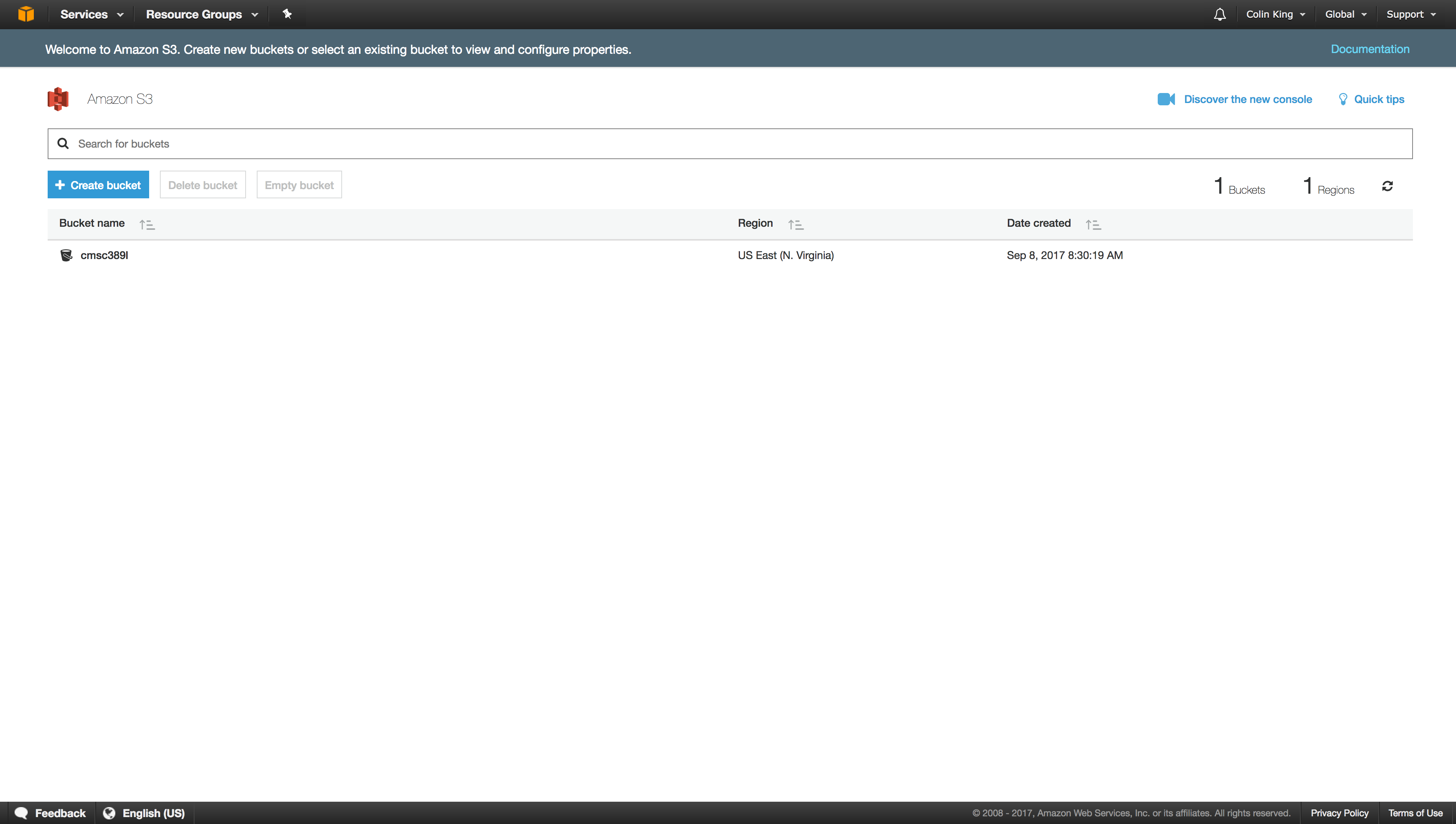This screenshot is from an Amazon S3 web interface. At the very top, there is a dark grey toolbar. On the far left of this toolbar, there is an orange cube icon. To the right of the cube, there is a drop-down menu labeled "Services" in white text, followed by another drop-down menu labeled "Resource Groups" in white text. To the right of "Resource Groups," there is a small, indistinct icon. On the far right of the toolbar, there is a bell icon. Proceeding rightwards, there appears to be a user name, possibly "Celine King," though the text is too small to read clearly. Next to the name, there is a drop-down menu labeled "Global," followed by another drop-down menu labeled "Support."

Beneath this toolbar is a lighter grey bar spanning the screen's width. On the left side of this bar, in white text, it says, "Welcome to Amazon S3. Create new buckets or select an existing bucket to view and configure properties." On the far right of this bar, "Documentation" is written in a very light blue text.

Below this grey bar, the background changes to white. There is an icon resembling a three-dimensional structure with three burnt orange dots stacked vertically, resembling walls and floors, positioned to the left of the text "Amazon S3."

A search bar runs horizontally across the screen. On the far right of the search bar, there are two icons: a camera with the text "Discover the new console" and a lightbulb with the text "Quick Tips."

Beneath the search bar, there are three tabs in the following order: "Create Bucket" (blue), "Delete Bucket," and "Empty Bucket." Below the tabs, the text "Bucket Name" appears, followed by the mention of a bucket name. The name appears to be something like "York" or "Greta," though it's very small and difficult to read clearly.